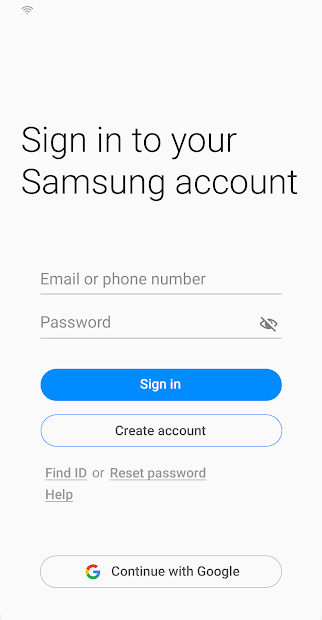The image is a screenshot of a Samsung account login page set against a plain white background. At the top, there is text prompting the user to "Sign into your Samsung account." Below this, there are two input fields: the first labeled "Email or phone number," represented by a horizontal line within a box; and the second labeled "Password," which includes an icon of an eye with a slash through it to indicate password visibility toggle. 

Under the password field, there is a prominent blue button with white text that says "Sign In." Beneath this, there is a white button with black text that reads "Create Account." Further down, in smaller gray text, are the options "Find ID" and "Reset Password Help." At the bottom of the screen, there is another white button, this time indicating "Continue with Google," accompanied by the Google 'G' logo on its left side.

In the top left corner of the image, a Wi-Fi symbol is visible, indicating connectivity status. The overall design is minimalist, with a primary focus on the text and buttons on the white background.